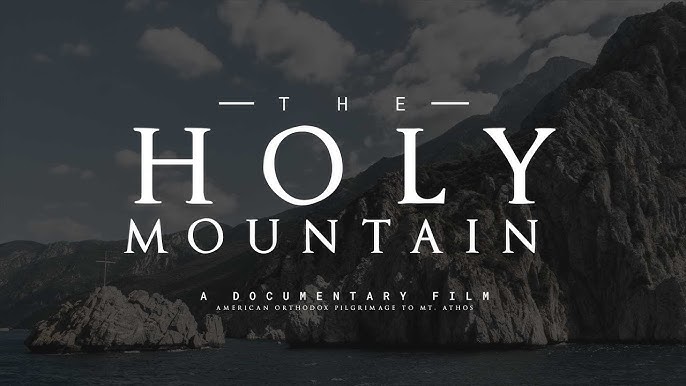The cover image for the DVD titled "The Holy Mountain" features a dark, dramatic landscape. Dominating the background is a large, rugged stone mountain that rises from the left to the right, disappearing off the top of the image, with another peak faintly visible in the distance. The foreground includes what appears to be a body of water, framed by more rocky terrain. The sky above the mountain is a deep blue with scattered white clouds, adding to the overall dark and moody atmosphere of the scene.

The main title text is set in striking white font. At the top, "T-H-E" is flanked by dashes, placed above the larger "H-O-L-Y" which is in all capital letters and spreads out to match the width of "MOUNTAIN" below it. Smaller text underneath reads "a documentary film," and further below is the subtitle "American Orthodox Pilgrimage to Mount Athos" in still smaller white print. The entire composition combines to create a sense of depth and solemnity, fitting the documentary's theme.